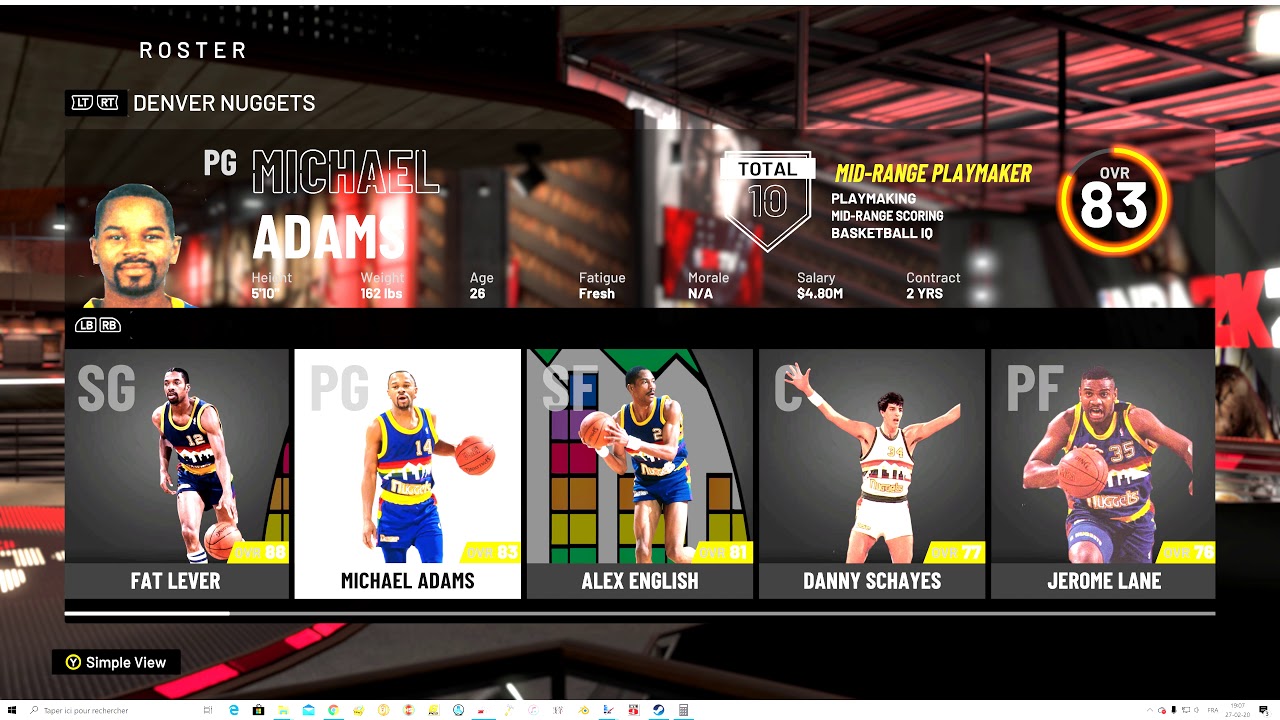The image appears to be a detailed roster screen, likely from a sports video game, showcasing the Denver Nuggets basketball team against a stadium background. The background, though partially obscured and difficult to discern, seems to feature a stadium with shifting color schemes: black and gray on the upper left, red and gray on the upper right, black on the bottom right, and a purple-gray hue on the bottom left. 

A prominent black rectangle contains various symbols and the text "Denver Nuggets." Below this, a player graphic labeled "PG Michael Adams" is displayed with small, unreadable white text underneath. To the right, more small white text is present but also unreadable.

The screen features a unique design element: a square that transitions into a triangular shape outlined in white with the text "Total 10" and the descriptor "Mid-Range Playmaker" beneath it in small, unreadable font. There is also an almost complete, orange-yellow circle with the text "OVR 83."

The roster details several players:
- SG Fat Lever, with an image of the player holding a basketball.
- PG Michael Adams again.
- SF Alex English.
- C Danny Schayes.
- PF Jerome Lane.

Each player's title is accompanied by their respective position and an image, contributing to the comprehensive presentation of the team's roster.